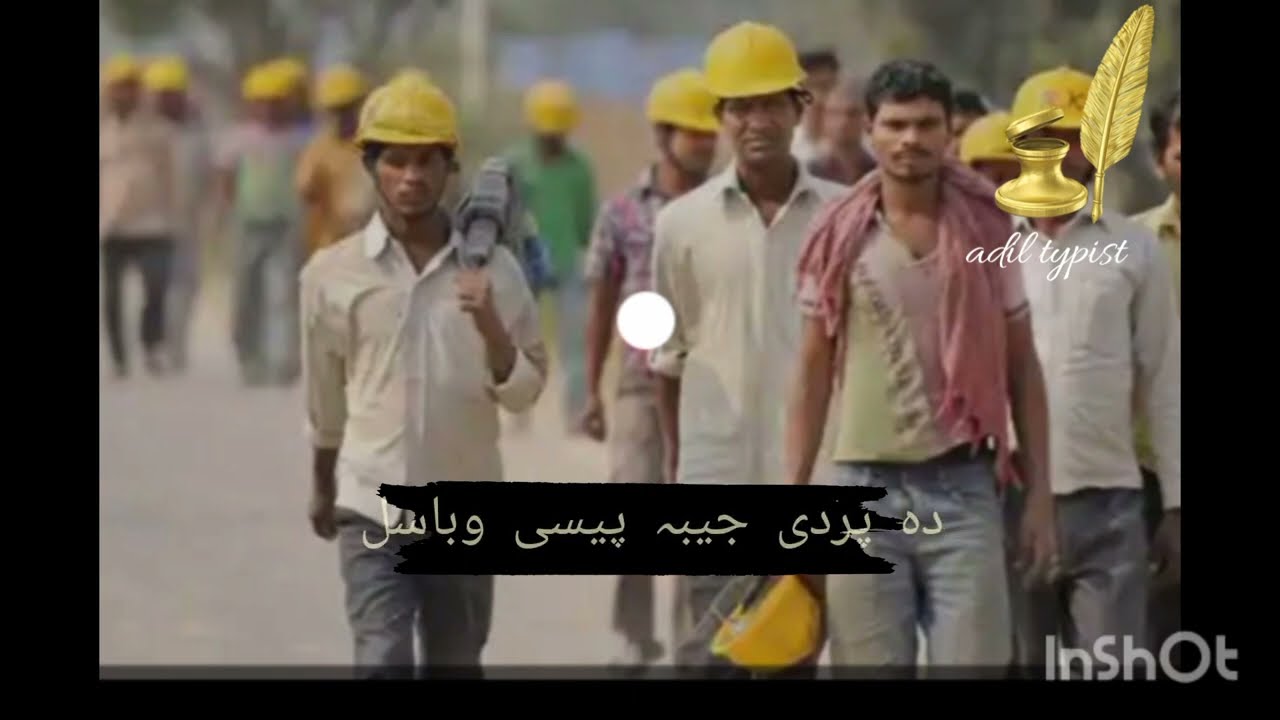The image depicts several Indian men walking, many of them donning yellow hard hats, except for one man who holds his hard hat by his side. Most of the men wear button-down collared long-sleeved shirts paired with jeans, while the man without the hard hat sports a different shirt and has a red scarf draped over his shoulders. The focus is on three men in the center, with one carrying a tool slung over his shoulder, while the rest of the crowd is blurry. At the top right, a feathered quill and inkwell icon accompany the cursive text "Adil Typist" in white. The bottom edge features a black rectangle with uneven sides, housing Arabic script, and overlapping text extending outside its bounds. The bottom right corner displays the word "InShot" in gray, partially transparent text.